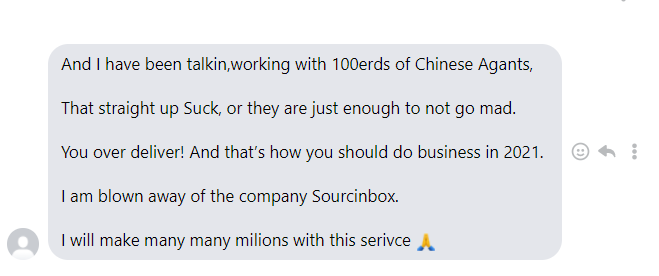In the provided image, a cropped screenshot of a chat is depicted. The chat bubble is gray, suggesting a simple and unobtrusive design. To the left of the chat bubble, there is a generic circular profile picture, displaying a gray background with a white person icon, indicating the user has not customized their profile image.

To the right of the chat bubble, several interactive icons are aligned vertically. At the top is a gray smiley face emoji icon, intended for accessing additional emojis. Just below the smiley face, there is a share icon, represented by an arrow pointing to the left, facilitating the sharing of the message. Finally, at the bottom, there is a menu icon offering additional options.

The message within the chat bubble reads as follows, though the text contains several errors and informalities:

"And I have been talking, working with hundreds of Chinese agents that straight up suck, or they just not enough to not to go mad. You over-deliver, and that's how you should do business in 2021. I am blown away by the company's source inbox. I will make many, many millions with the service." This message concludes with a praying hands emoji, indicating gratitude or a hopeful sentiment.

Note: The original message contains several typing errors, such as "100 herds" which is likely intended to be "hundreds," and "A-G-A-N-T-S" which should be "agents." The phrasing also suggests that English may not be the writer's first language, leading to some structural inaccuracies.